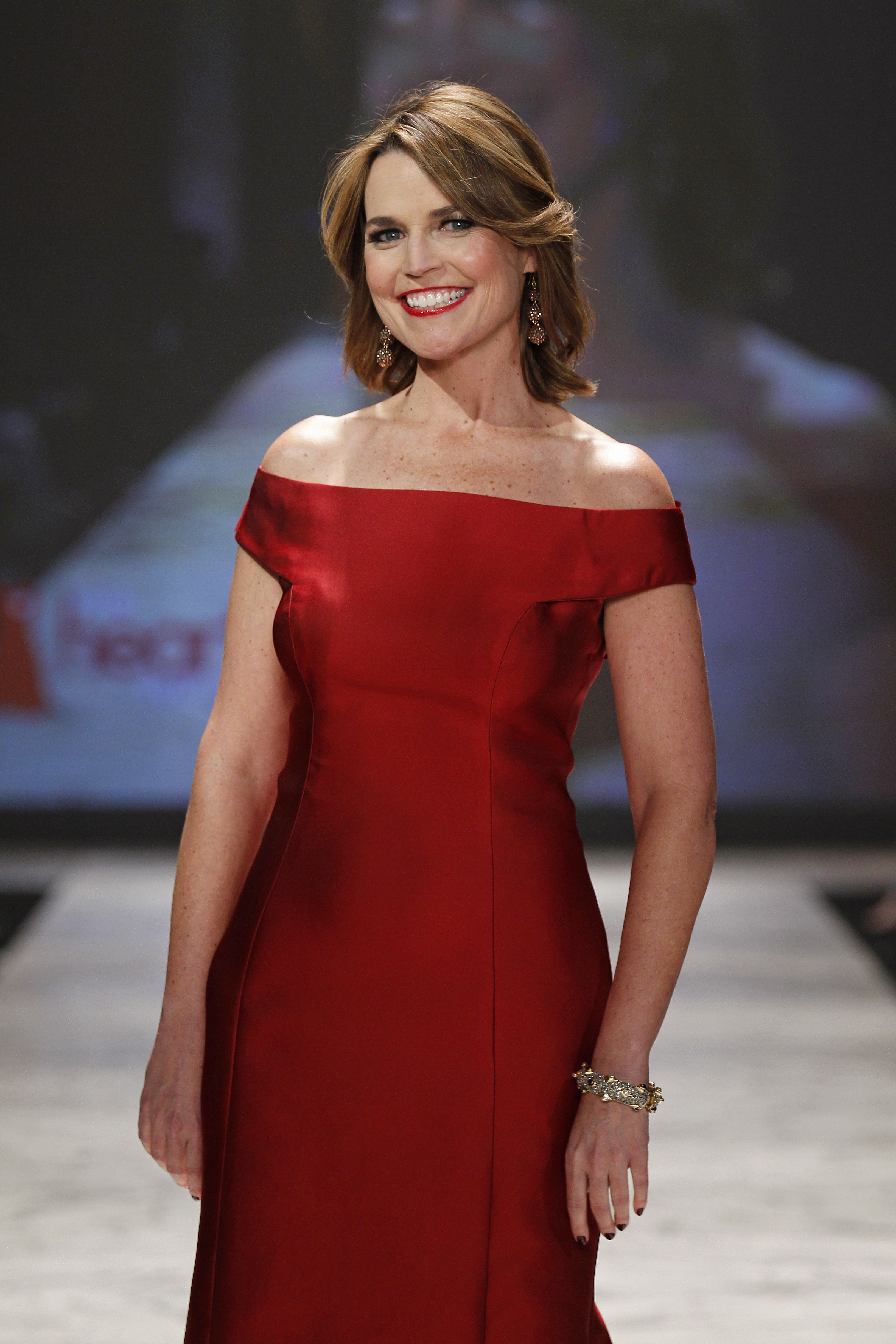This photograph captures a striking young Caucasian woman standing confidently on a white runway stage. Centered in the frame, she exudes elegance with her light brown hair, parted slightly to the right and cascading just above her shoulders. Her flawless professional makeup, highlighted by red lipstick, accentuates her radiant smile. She wears a sophisticated strapless red gown, adorned with shoulder caplets that drape over her bare upper arms, emphasizing her formal and poised stance. Her right arm is relaxed and straight by her side, while her left arm is slightly bent at the elbow, showcasing a heavily bejeweled gold bracelet. The background features a stage setup, possibly with a video screen, reinforcing the runway context of the scene.